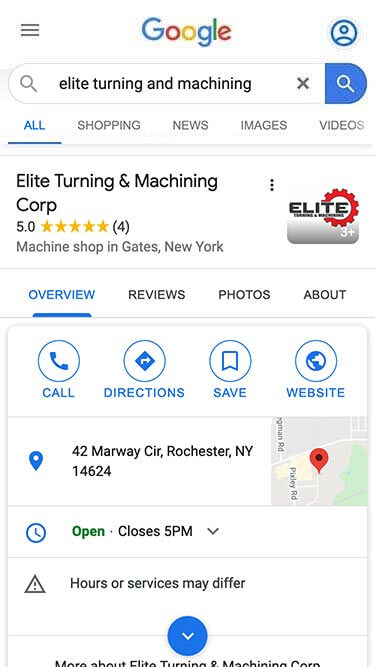This image captures a screenshot of a Google search result for "Elite Tuning and Machining Corp." The background is white with the Google logo prominently displayed at the top center. In the top right corner, there is a blue and white user profile icon, while the top left corner features a menu button that opens additional options.

Below the Google logo is the search bar, containing the query "Elite Tuning and Machining." Underneath the search bar, there are various tabs including "All," "Shopping," "News," "Images," and "Videos." The primary search result highlights "Elite Tuning and Machining Corp," and its logo appears on the right side, featuring black, white, gray, and red colors. Three additional thumbnail images accompany the logo, with a "+3" symbol indicating more images are available.

The search result notes that the company has four reviews, boasting a perfect 5.0 rating. It identifies the business as a machine shop located in Gates, New York. Below this information, multiple tabs are displayed, including "Overview," "Reviews," "Photos," and "About." Users have options to call the company, get directions, save the listing, or visit the official website. Additionally, the business's address, its closing time of 5 p.m., and the note that it is currently open are provided, along with a disclaimer that hours or services may differ.